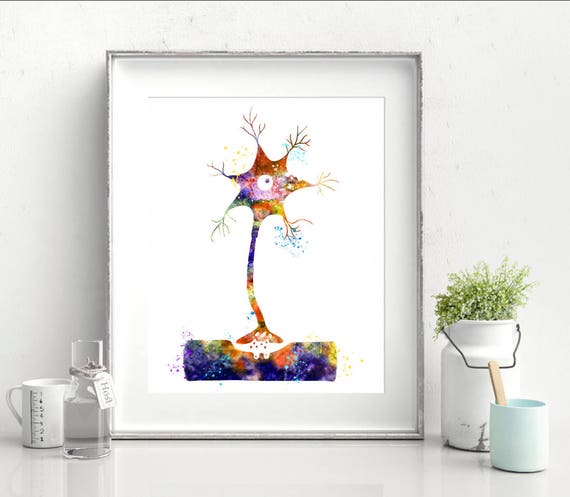The image features a framed abstract painting with a thin silver frame and white matting, leaning against a very light gray, almost white wall. The painting itself is vibrantly colorful, predominantly featuring purple, dark blue, orange, yellow, pink, green, and red. The abstract design depicts a plant-like structure that emerges from a cylindrical base, growing into a seven-pointed star shape with branches and an eye-like white circle with a dark dot in the middle. Surrounding the framed picture on the floor are several objects. To the left of the painting, there is a white tea mug with black measurement lines and a clear glass filled halfway with water. On the right side, there is a slightly taller white jug containing a house plant and a pale blue cup with a wooden stick protruding from it. The overall composition gives the impression of viewing the scene from about five feet away.